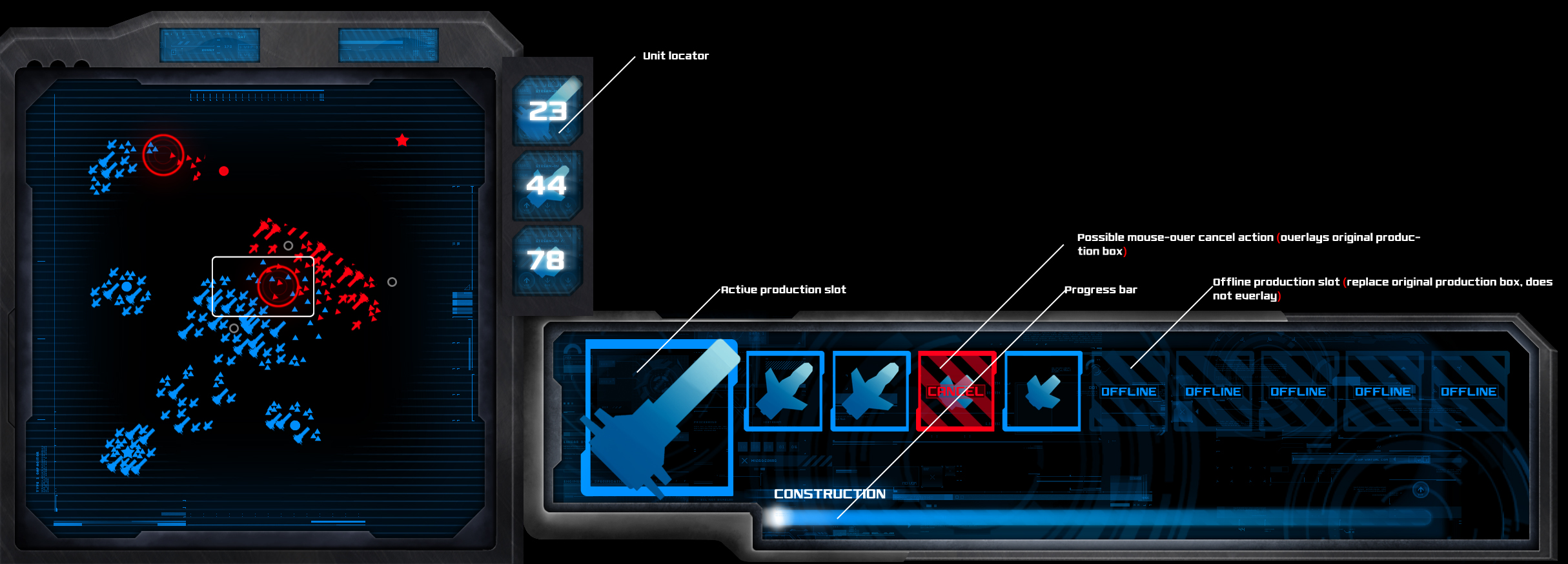This is a long, rectangular photograph resembling a screenshot from a computer game, displayed on a machine's futuristic-looking screen. The screen, set against a black background with white text and blue and red icons, portrays various elements that converge into a detailed battle scene. 

On the left side, there's a radar-like display showing blue and red aircraft-like characters engaging in combat, highlighted within a red circled area, giving the impression of an active battle. Surrounding the radar screen are numerical indicators, including white numbers such as 23, 44, and 78, possibly representing unit counts or other significant metrics.

To the right, a second section contains descriptive boxes presenting detailed diagrams and explanations of each unit involved in the fight. Notable elements include four blue weapons, with one especially large weapon, and a third weapon marked with a red cross, indicating its status. Further down, there are smaller blue boxes labeled "off-line," and a progress bar under the label "construction." Arrows and small white text point to each symbol, providing additional context and details that are slightly challenging to discern. This composition, with its intricate details and highlighted battle scenarios, strongly suggests the screenshot belongs to a strategy or combat video game.